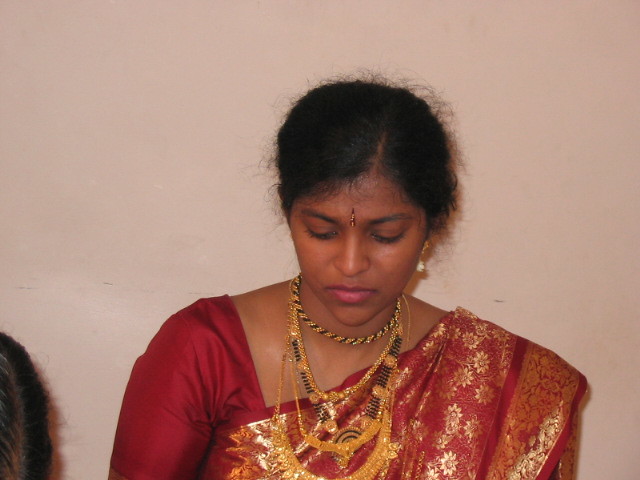The image is a horizontal rectangular photograph of an Indian woman seated against a beige wall, with the focal point being her upper body from chest up. She wears a traditional red and gold satin sari, adorned with floral designs, which drapes elegantly over her shoulder. Her dark hair, parted slightly off-center, is swept back into a bun or braid. She features a solitary gem centered on her forehead between her eyebrows, hinting at cultural significance, and she dons white, dangling earrings that contrast her bare makeup look. Around her neck are multiple gold necklaces of varying lengths and black details, adding to her intricate ornamentation. The woman gazes downward with a sober expression, suggesting contemplation. In the bottom left corner of the image, a sliver of another person, identifiable only by a dark shoulder and head, peeks into the frame, emphasizing the woman as the main subject.